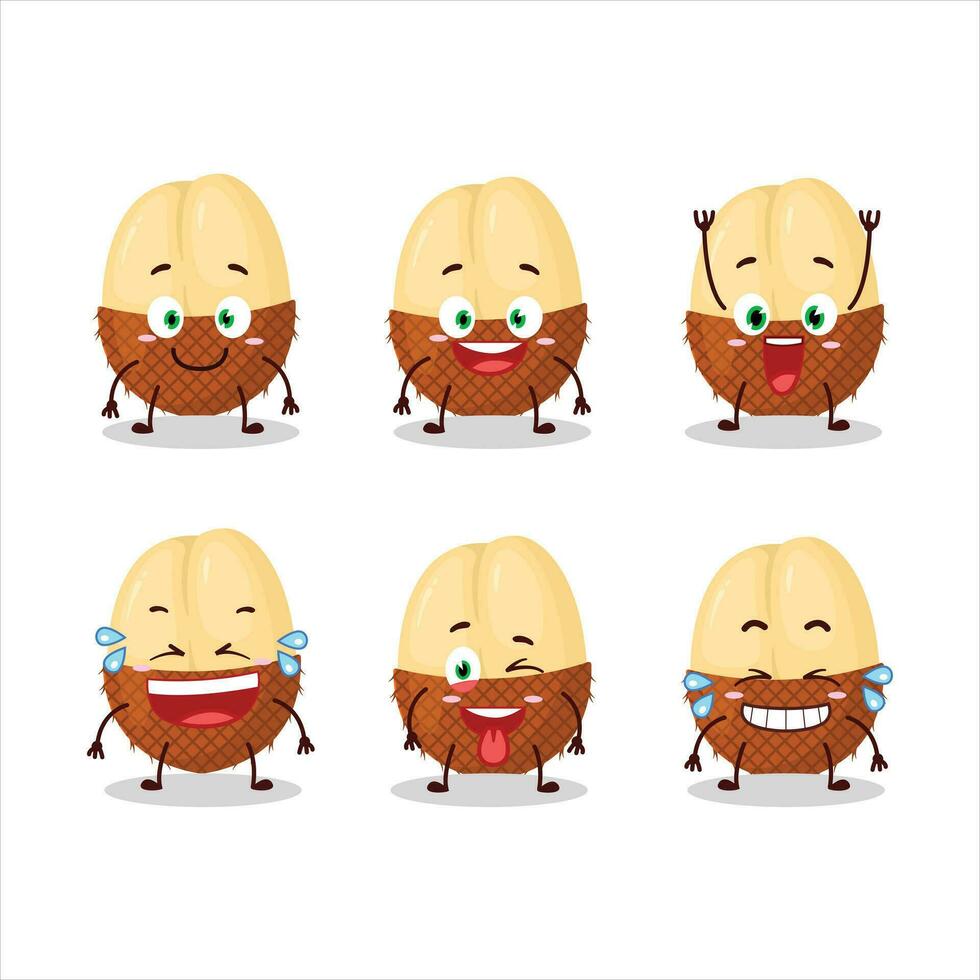The image features a set of six cartoon-style anthropomorphized peanuts, each exhibiting a different facial expression and emotion. The peanuts are characterized by a tan, light brown upper half and a darker brown, crosshatched lower half resembling an unpeeled shell. Each peanut has stick-like arms and legs, green eyes with raised eyebrows, and small pink blushes on their faces.

From left to right, the top row peanuts portray the following emotions:
1. A happy peanut with a closed smile and green eyes.
2. A surprised peanut with its mouth open.
3. An excited peanut with its arms raised and mouth wide open, as if experiencing a thrill.

In the bottom row, the peanuts display these expressions:
1. A laughing peanut with its mouth open, eyes closed, and tears of joy streaming down.
2. A playful peanut winking with one eye closed and sticking out its tongue.
3. A smiling peanut with tears of laughter, showing a full set of teeth.

Each animated peanut is set against a simple shadow backdrop to give a sense of depth. The detailed faces and expressive features capture a wide range of emotions, bringing the inanimate peanut characters to life.